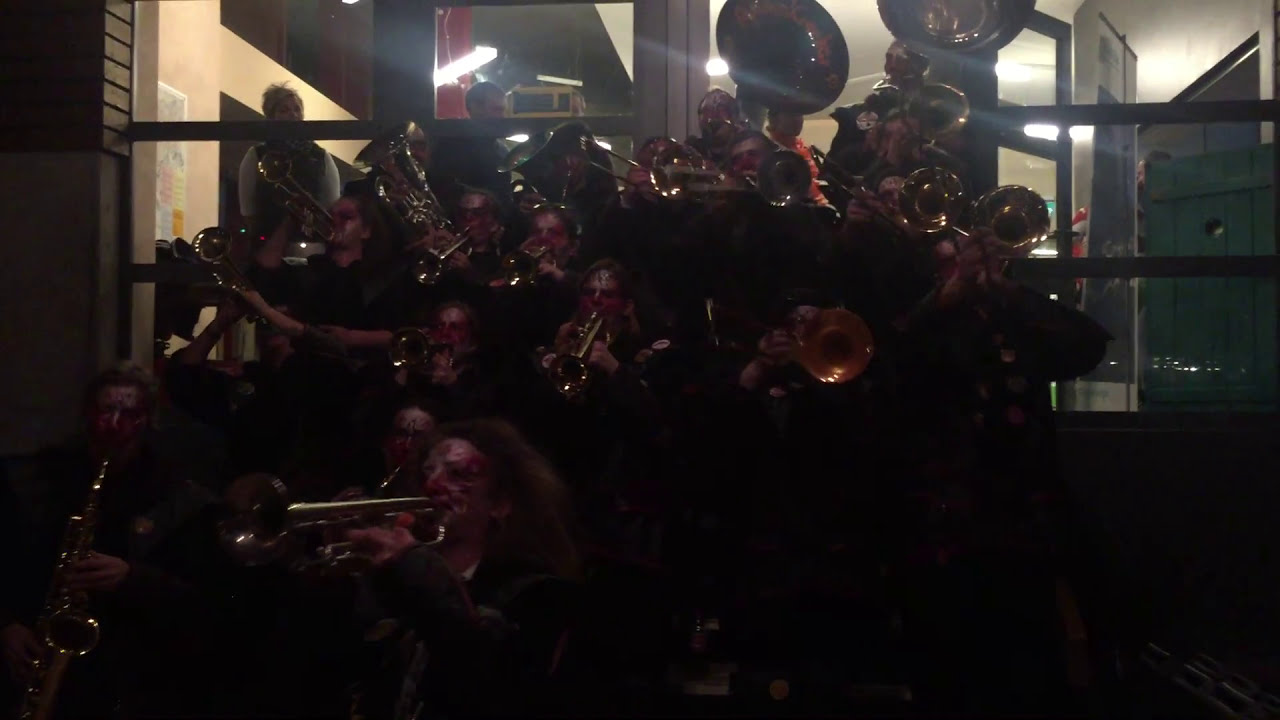The image showcases an orchestra performing at an event, seemingly staged on steps or a slightly elevated platform. The poorly lit scene makes it difficult to discern specific details or the exact number of orchestra members, who are predominantly playing brass instruments such as trumpets, saxophones, trombones, and tubas. Dressed in black attire, the musicians' faces are adorned with makeup designed to evoke a horror or zombie theme, featuring elements like red paint. The backdrop includes a glass window or wall, behind which a well-lit area reveals onlookers observing the performance. These spectators are positioned within an adjacent, more illuminated section of the venue, contrasting sharply with the dimly lit orchestra.